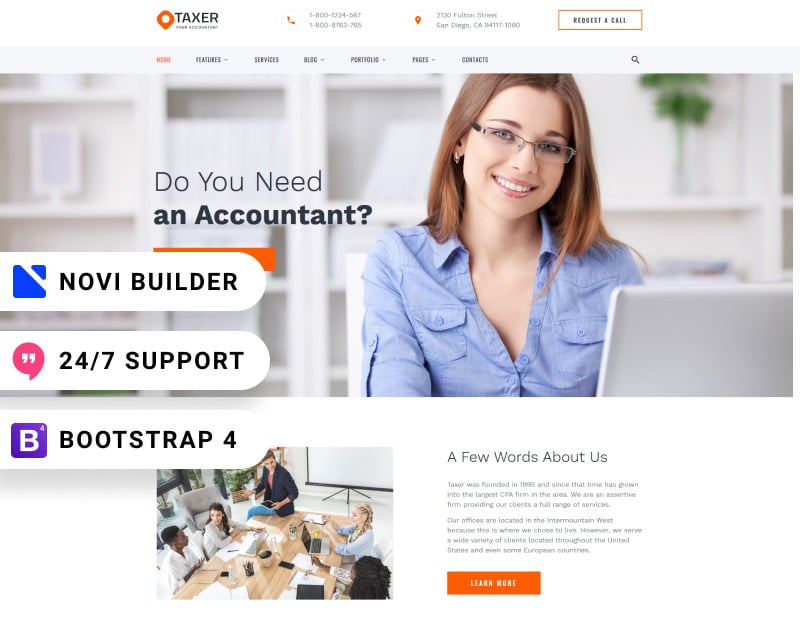The website interface prominently features the company name "Taxer" positioned at the top left corner, accompanied by an orange diamond-shaped logo with a white circle in the center. Situated to the right of the logo, there are two contact phone numbers indicated by an orange phone icon, and an orange location pin symbol displays the address. Adjacent to these details is an orange-bordered rectangular button with a white interior, labeled "Request a Call." 

Below this section lies the website's navigation menu, presented in light gray. This menu includes clickable black text options such as Home, Features, Services, Blog, Portfolio, Pages, and Contact. A search bar is conveniently located on the far right.

The main visual on the homepage features a professional woman with brown hair, a white complexion, and black glasses, smiling warmly at the camera. She is clad in a blue button-down shirt and is seated at a desk with a computer in a predominantly white office setting. A black text overlay across the image reads, "Do you need an accountant?". To the left of this text, bullet points highlight features like "Nobie Builder," "24-7 Support," and "Bootstrap 4."

Beneath the primary image is a secondary section with a photograph of five individuals engaged in a discussion around a light wood table, with a projector screen visible in the background. This section is captioned "A Few Words About Us" and provides a brief history of Taxer. Founded in 1995, the firm has grown to become the largest CPA firm in its area, offering a comprehensive range of services. Their primary office is located in the Intermountain West, but they cater to clients across the United States and in several European countries. Below this narrative, an orange box labeled "Learn More" invites further exploration of their services.